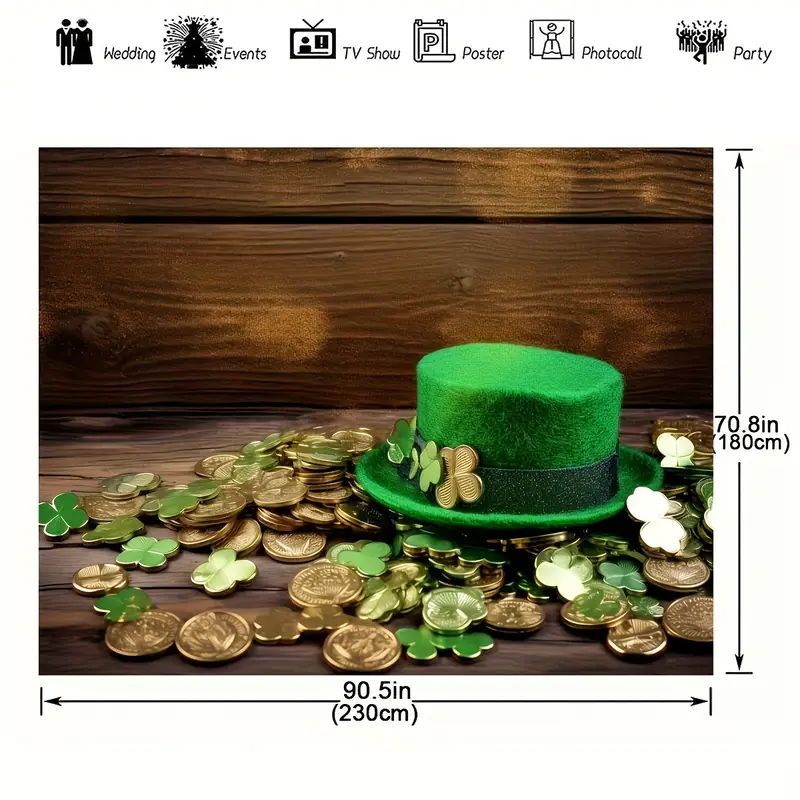This is an image, most likely a photograph, featuring a green St. Patrick's Day hat positioned slightly to the right side on a wooden, slatted surface that might be a table or bench. The hat appears to be made of wool felt or a furry material and is adorned with a dark green satin band. The band is further decorated with various shamrocks and four-leaf clovers in shades of dark green, mint green, and gold. Surrounding and underneath the hat are numerous coins, mostly bronzy yellow or silver, mixed with additional clovers. Dimensions of the image are provided along the right side and bottom, indicating it measures 90.5 inches (230 centimeters) in length and 70.8 inches (180 centimeters) in height, adding a technical aspect to this festive, detailed representation of St. Patrick's Day elements.